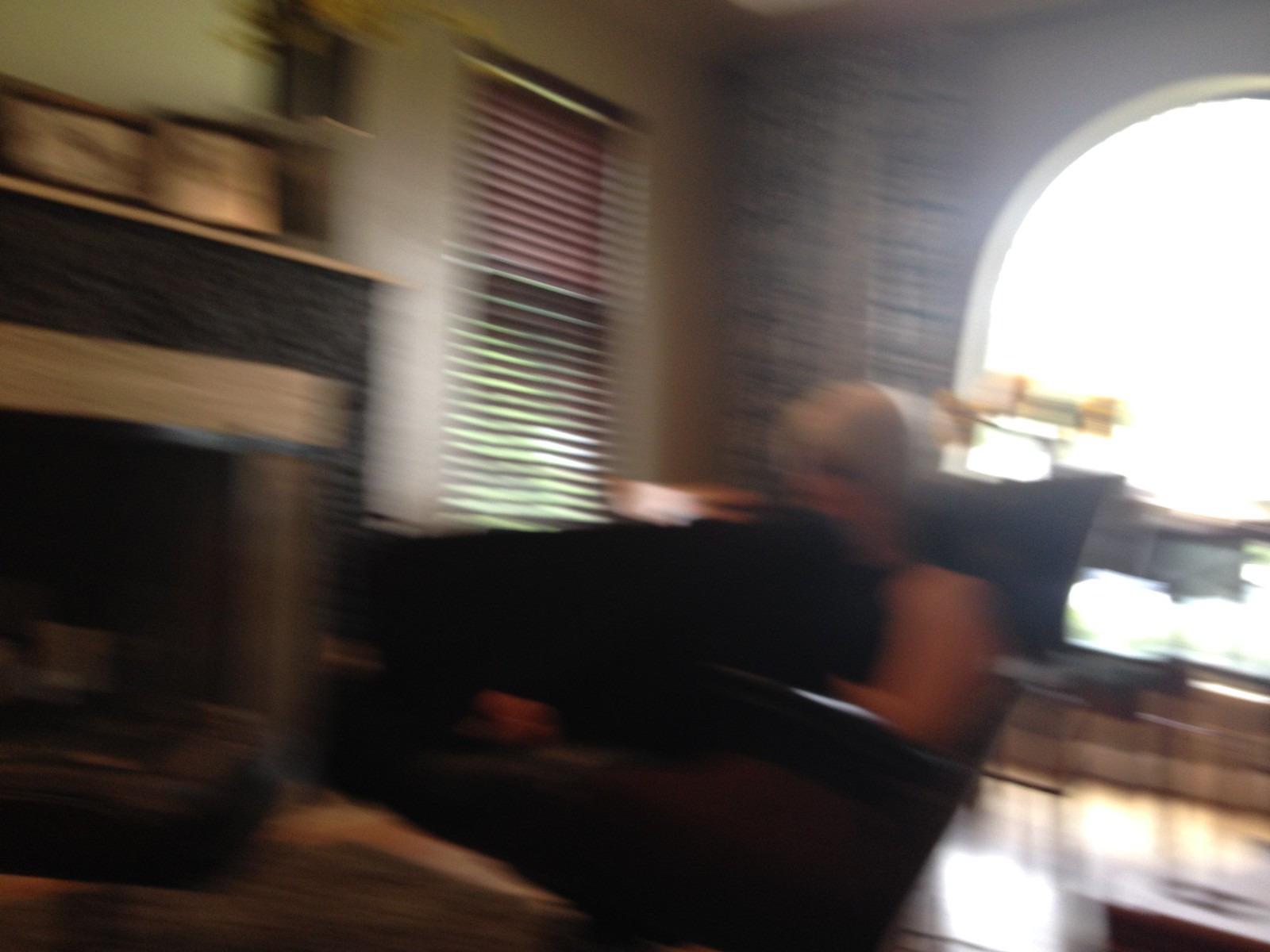In this warmly lit photograph taken inside a cozy home, a woman with blonde hair sits in a large, comfortable chair, her legs possibly crossed and her body leaning slightly back. She is oriented towards the left side of the image. To her immediate left, a fireplace emanates a gentle warmth, while a window adorned with maroon blinds is positioned on the right side of the fireplace. Behind her to the right, a large arched window allows an abundance of natural light to flood into the room, casting a soft glow on the scene. Though the image is blurry, it appears that a large black dog is nestled in her lap, adding a touch of companionship and contentment to the serene atmosphere.